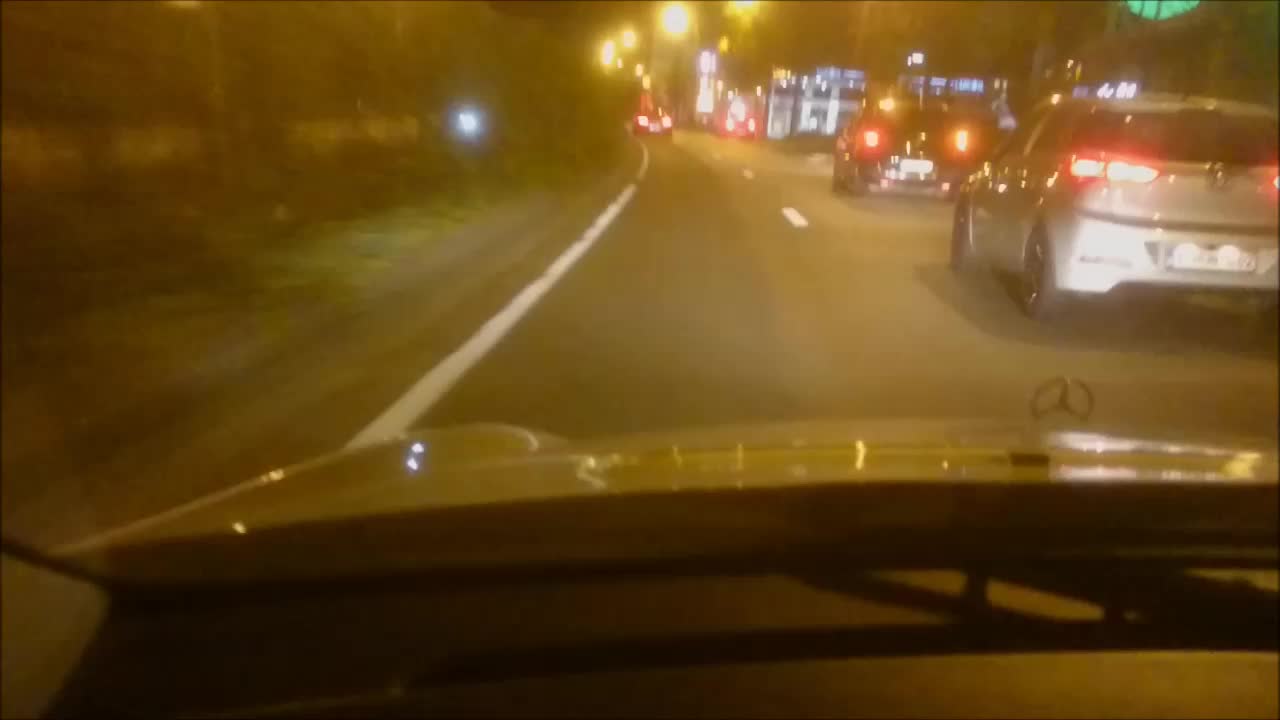This vivid color photograph, taken at night from inside a white Mercedes-Benz in the left lane of a two-lane highway, captures the driver’s view through the windshield. The scene unfolds under the glow of streetlights, showing a busy road with multiple vehicles. Ahead in the left lane, a car's brake lights are visible in the distance, indicating a stop. In the right lane, there are three cars: the nearest one is white, followed by a black car, and another further up the road with only its brake lights visible. The left side of the highway is bordered by a grassy field with a tree line, while the right side is lined with illuminated businesses and various street signs. In the distance, headlights from oncoming traffic suggest a well-traveled boulevard.